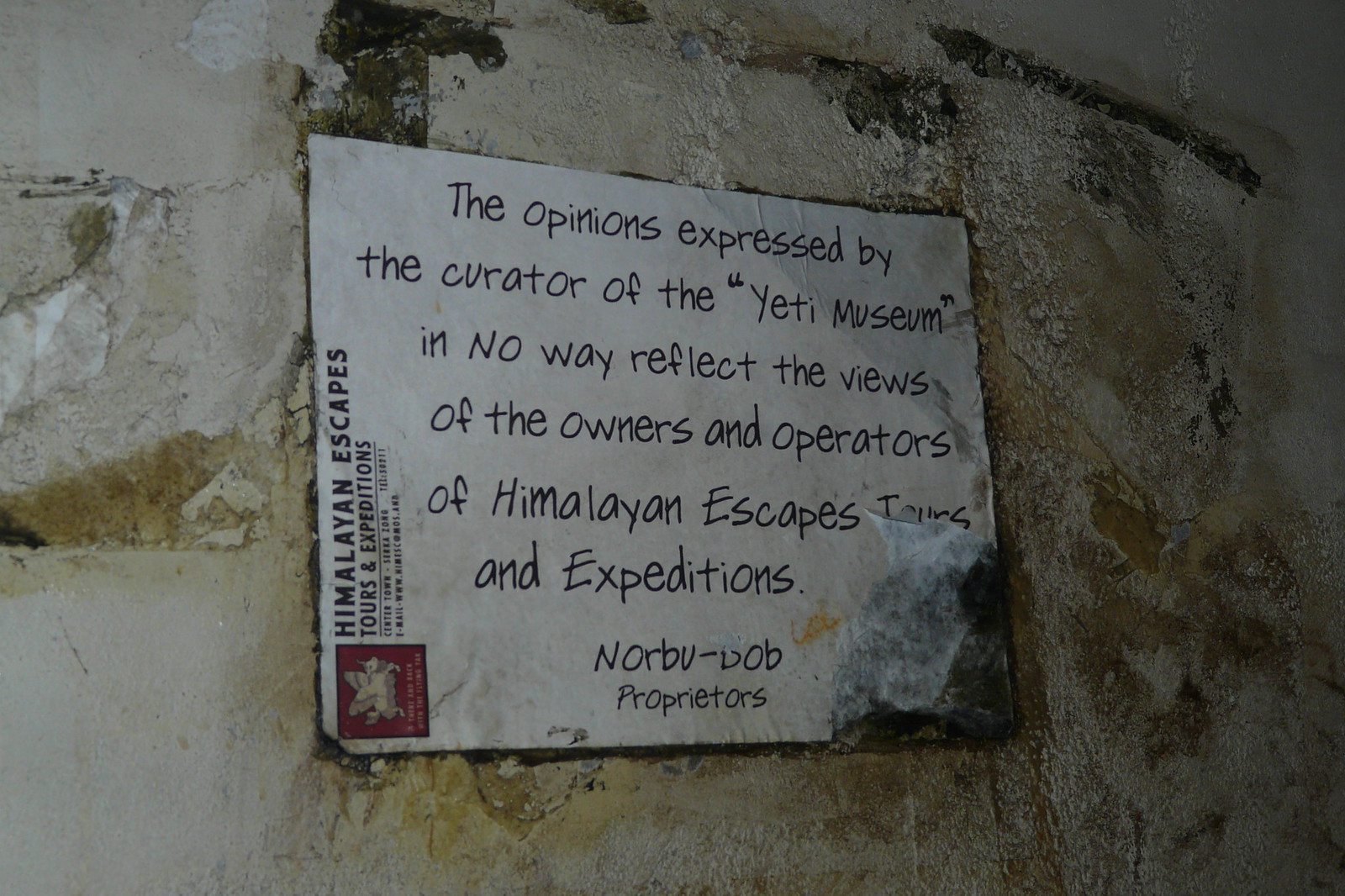An old and poorly maintained wall, once painted white but now peeling and stained with patches of yellow, gray, and black, serves as the backdrop. Adorning the wall is an equally worn and decayed white sign, notably distressed in the bottom right corner. The critical text on the sign states: "The opinions expressed by the curator of the Yeti Museum in no way reflect the views of the owners and operators of Himalayan Escapes, Tours, and Expeditions, Norabu-D.O.B. Proprietors." The sign features vertical text on the left side reading "Himalayan Escapes, Tours, and Expeditions," with additional small, unreadable text beneath it. In the bottom left corner of the sign sits a red square containing a yellow emblem, which appears to be a stylized image that is difficult to discern due to wear and positioning. The overall scene conveys a sense of neglect and age.